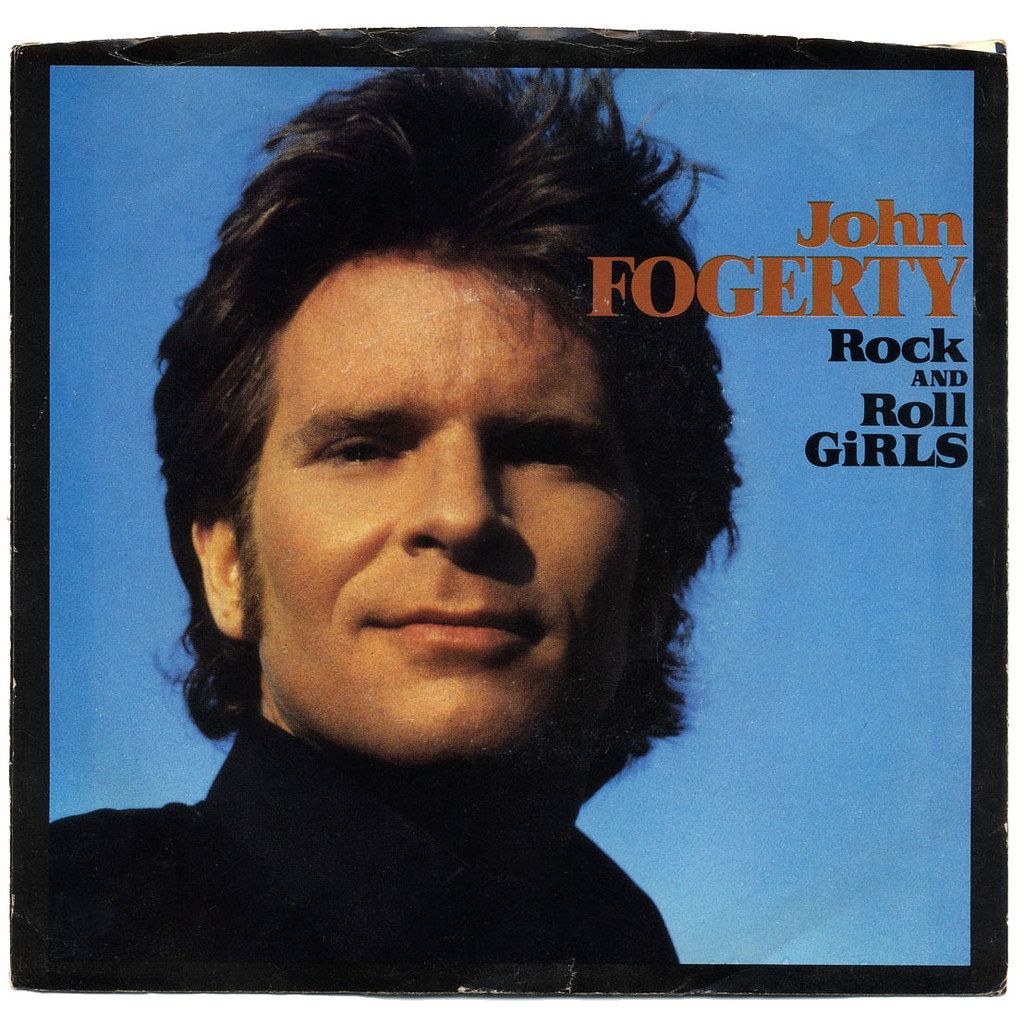The image is an album cover featuring John Fogerty, one of the founding members of Creedence Clearwater Revival. The cover has a sky-blue background suggesting an outdoor setting. John Fogerty is looking straight ahead at the camera. He has thick dark brown hair, longer sideburns, and dark eyebrows, with a clean-shaven face. He is wearing a black jacket or turtleneck. His name, "John Fogerty," is prominently displayed in orange text on the right side, while the album title, "Rock and Roll Girls," is written in black text below it. The cover is bordered in black and appears weathered, indicating it's been in a collection for some time. The emphasis is on the upper body of Fogerty, giving a focused and direct appeal to the observer. This detailed depiction is likely that of an LP or CD cover art.